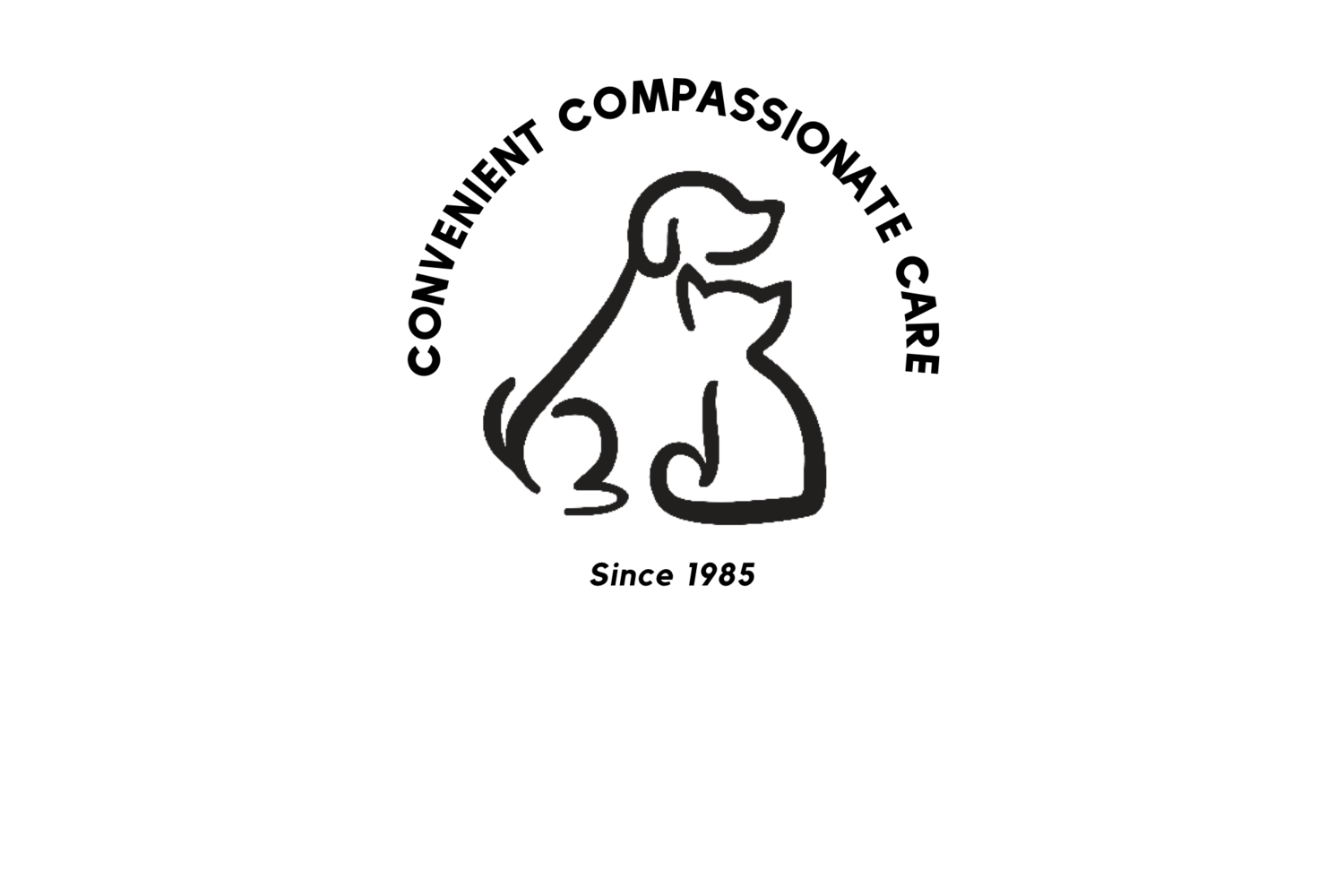The logo features a minimalist and timeless design with a white background and bold, black text. The words "Convenient, Compassionate Care" are written in an arch, forming a circular shape around the central image. Inside this circular text, there is an abstract, faceless silhouette of a dog and a cat melded together. The dog faces to the right while the cat faces to the left, creating a balanced and harmonious visual. Below the animals, the text "Since 1985" is prominently displayed. The simple, thick-lined design ensures that the logo has a timeless appeal, making it suitable for long-term use.